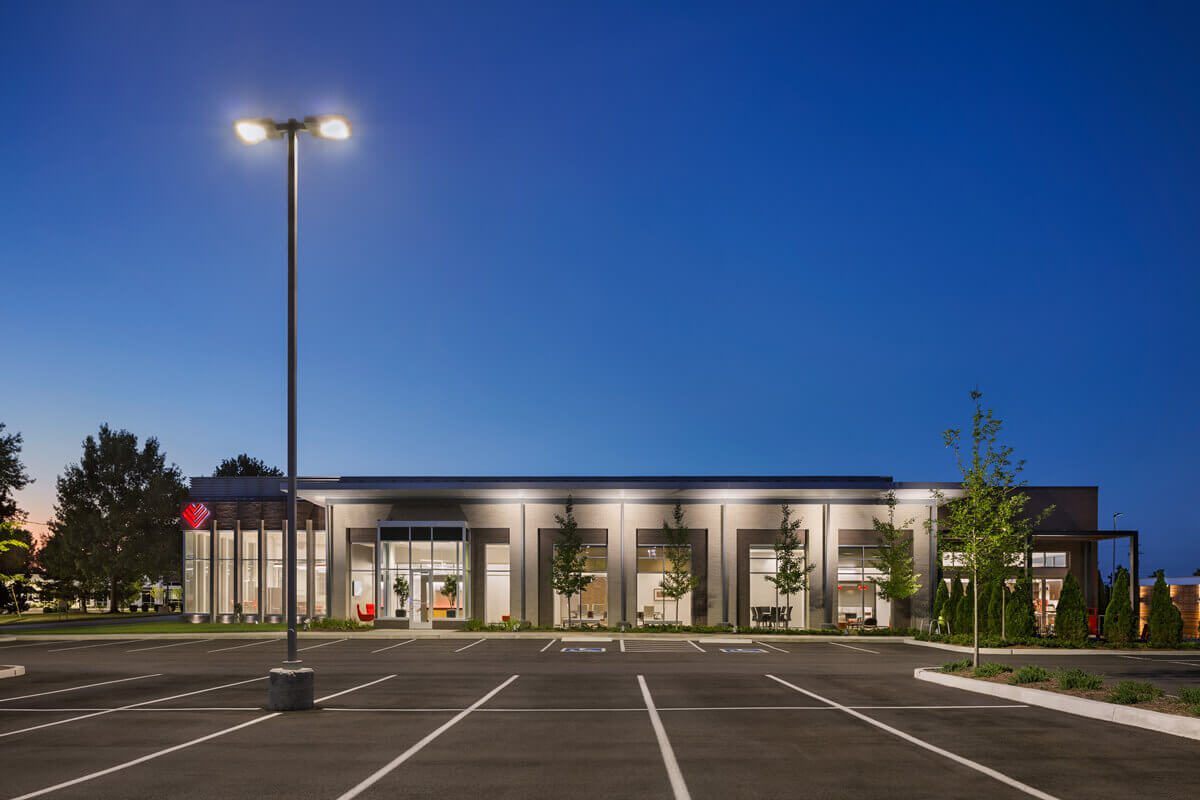This image captures an empty, freshly painted parking lot in the evening, with the darkening sky taking up about half of the frame. The parking lot, featuring crisp white lines on the black asphalt, has one lit street light on the left side providing some illumination. The building in the mid-ground appears to be a beige-brown or copper-colored one-story office or educational building, characterized by its square and flat structure with many windows. Through some of the windows, conference rooms or office setups can be seen, suggesting its use for professional or educational purposes. The property is well-landscaped with neatly manicured trees and plants scattered around the building’s vicinity, contributing to the modern aesthetic of the scene. Additionally, the sky transitions from blue to a hint of orange, indicating that the sun has recently set. A logo is visible on the building’s front, though it is not recognizable.